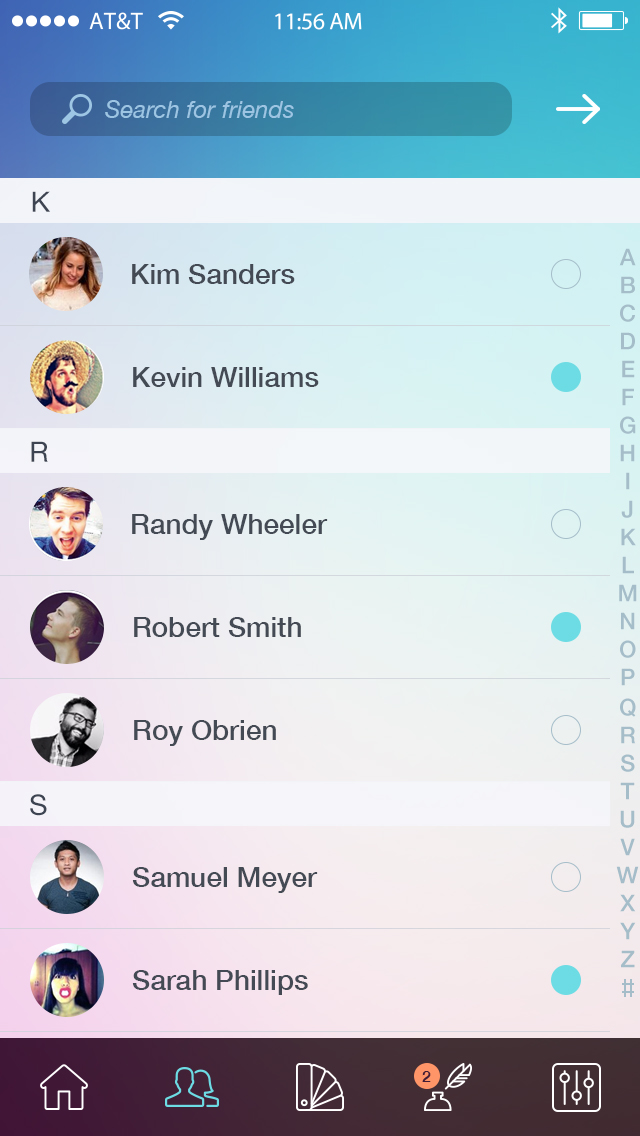The image is a rectangular snapshot taken from a cell phone, oriented vertically. At the very top, a bluish-turquoise border spans the width of the image, containing several icons and indicators. On the top left, five white circles display full signal strength next to the label "AT&T." Adjacent to this, a Wi-Fi symbol also shows full strength. Centered at the top, the time is displayed as "11:56 AM." On the far right, there are icons for Bluetooth and a battery, which appears to be about three-quarters charged.

Beneath this border, there's a darker blue box with faint text, featuring a search bar labeled "Search for friends" alongside a magnifying glass icon. To the right of the search bar, there's a right-pointing arrow.

The main content of the image displays a list of contacts organized alphabetically. The first section is demarcated by a white border containing the letter "K," under which two contacts, "Kim Sanders" and "Kevin Williams," are listed, each accompanied by respective profile pictures. 

The next section, marked by a banner with the letter "R," includes three contacts: "Randy Wheeler," "Robert Smith," and "Roy O'Brien," again with corresponding profile pictures. 

Following this, another banner displays the letter "S," listing two more contacts: "Samuel Meyer" and "Sarah Phillips," each with their profile pictures.

At the bottom of the image, a border features several icons, though these are not described in detail.